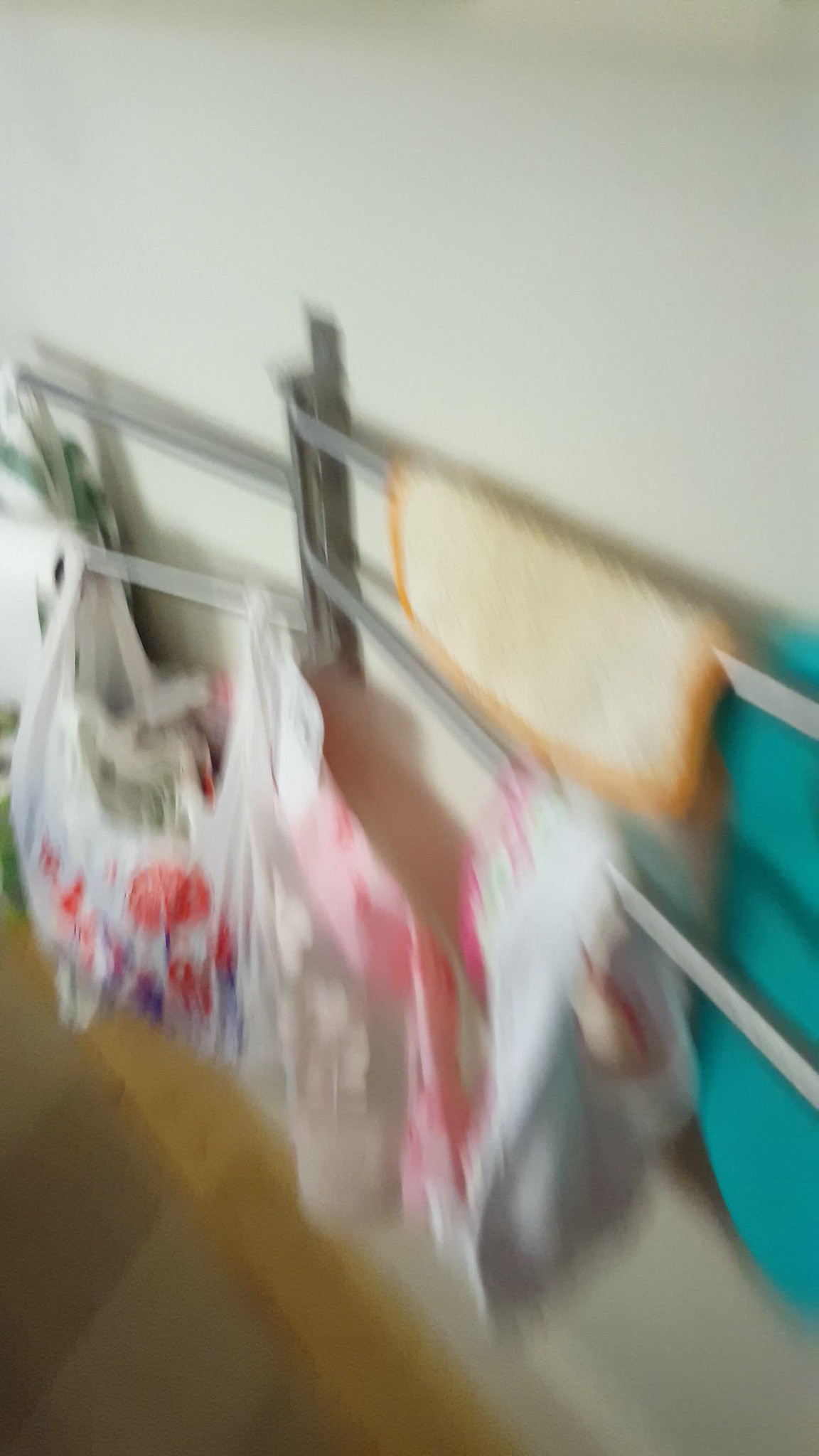This is a very blurry photo showing a clothesline-like rack system attached to a white wall, likely outside a house. The rack, which appears to have a hinge mechanism, supports multiple metal rods extending outward. On the lower rod, several plastic grocery bags are hanging. To the right of the frame, there's a yellow cloth, and further to the right, a turquoise-colored cloth is also hung. An orange washcloth with a darker outline hangs on one of the racks, along with what seems to be a blue towel. The floor beneath is a brown wooden panel or similar surface. Visible on one of the rods is a toilet paper roll or possibly a paper towel roll. Despite the blurriness, the shadows cast by these items add depth to the image.